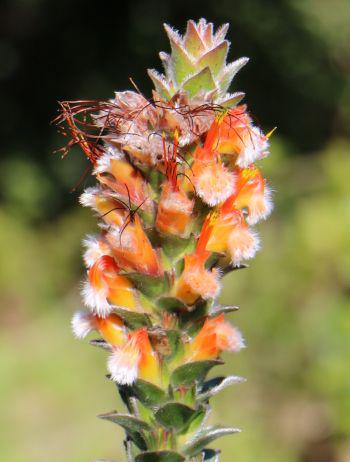This nature photo captures a close-up view of a Mementes, also known as Pagoda, an evergreen shrub. The image focuses on one of its distinctive buds. This crisp shot reveals the bud's interesting texture and color: small, orange-ish red petals with fuzzy white tips that transition into thin, hair-like red strands towards the top, which resembles a spiky green plant. The background, though filled with greenery, is out of focus, rendering the details indistinguishable and creating a blurred effect that contrasts with the sharpness of the bud. The upper part of the background appears black, further highlighting the vibrant colors and intricate design of the flower. Despite its cactus-like appearance, this plant lacks thorns or prickers. Some elements, like wire-like fuzziness and red stringy bits near the top, add unique texture to the photo. This outdoor shot, taken during daylight, captures the plant's natural habitat, emphasizing its rich colors and unusual features.